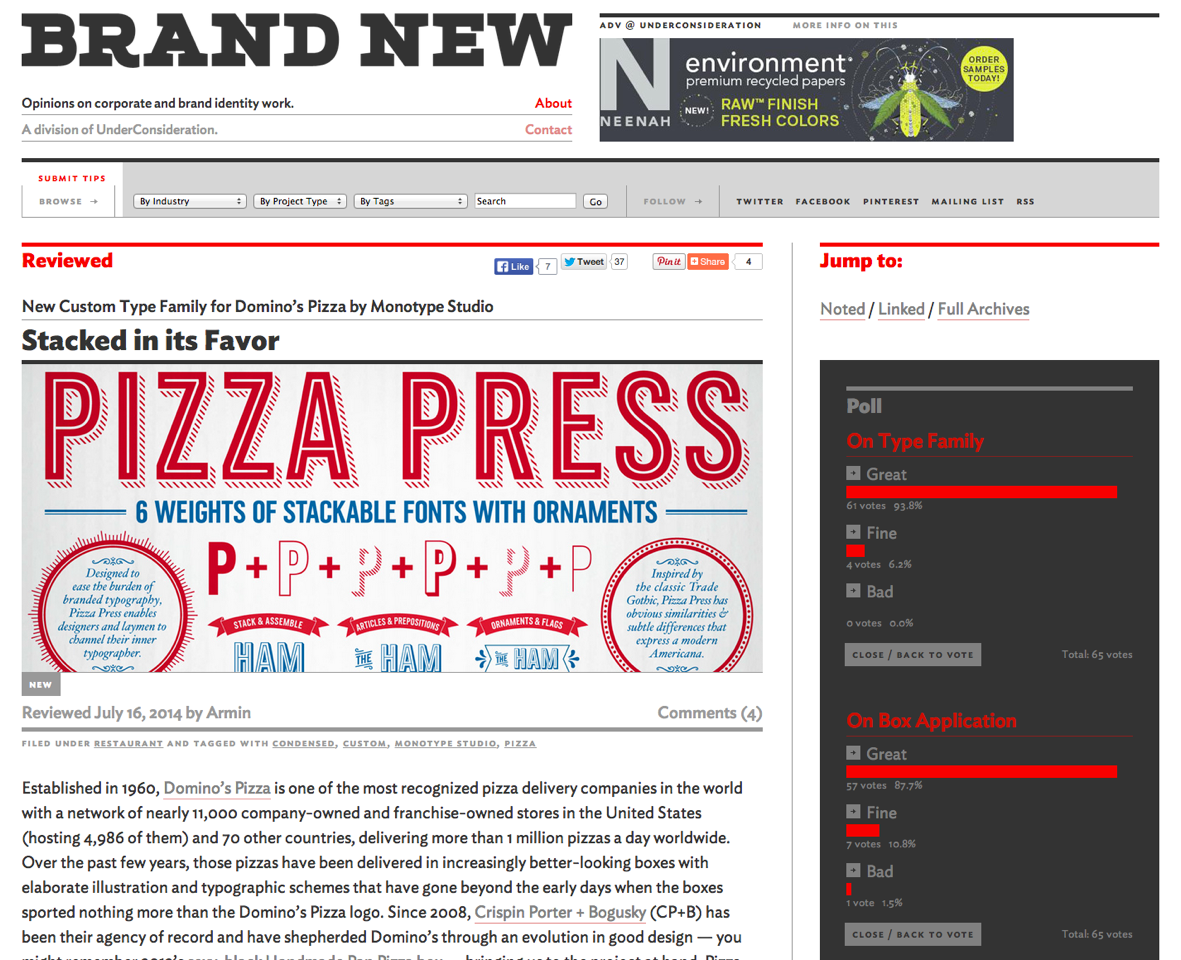The image is a screenshot of a website. At the top-left corner, the page prominently displays the phrase "Brand New" in large, bold black letters. Just below, it reads, "Opinions on corporate and brand identity work, a division of Under Consideration." 

On the top-right corner is presumably an advertisement, with the text: "Environment, premium recycled papers, raw finished fresh colors." Beneath this, in light gray text, it says, "Submit type." 

The website offers browsing options, including categories such as "by industry," "by project type," "by my tags," and a search function. Additionally, you can search the site through social media platforms like Twitter, Facebook, Pinterest, or join their mailing list.

The central focus of the webpage is an article titled "Pizza Press," showcasing six variations of stackable fonts with ornamentation. It states that the typeface was "reviewed" and reveals that it is a "new custom type family for Domino's Pizza by Monotype Studio." The visual display includes multiple 'P' letters, some solid and others outlined in red. There are also two red circles with blue text inside. Below this main section is a written paragraph that appears to discuss specifics about Domino's Pizza.